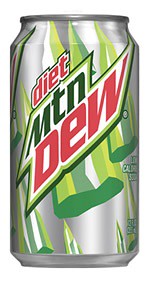The image features a can of Diet Mountain Dew against a pure white background, presenting a clean and unobstructed view of the can itself. The cylindrical container prominently exhibits a metallic silver finish on both the top and bottom sections. The main body of the can is also primarily silver, adorned with a dynamic striping pattern composed of lime green, hunter green, and white hues. These stripes converge to form a design reminiscent of mountain peaks.

Centrally displayed, the product’s name reads "Diet Mountain Dew." The word "Diet" is in lowercase and colored red. The abbreviation "MTN" for "Mountain" is rendered in dark green, while the word "Dew" is prominently capitalized and also colored red. The precise and bold typography, combined with the vibrant color scheme, effectively captures the essence of this iconic beverage.